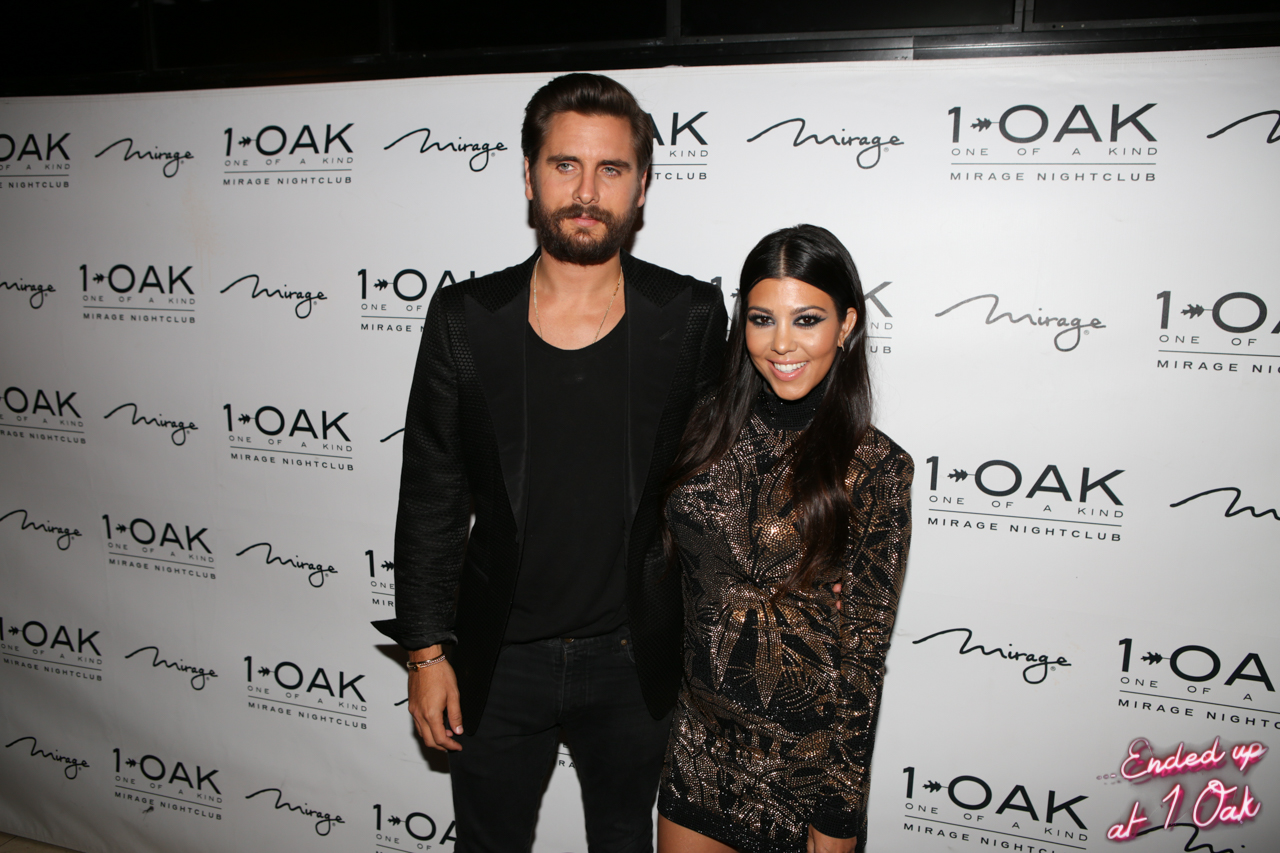In this image, the celebrity couple Scott Disick and Kourtney Kardashian pose against a white backdrop repeatedly adorned with the cursive script "Mirage," alongside "One Oak" and "One of a Kind Mirage Nightclub." Scott, on the left, is dressed in a shiny black jacket over a black T-shirt and jeans, accessorized with a bracelet on his right arm. He has short dark hair, blue eyes, and a short beard, and his gaze is directed slightly to the right. Kourtney, standing next to him with his arm around her, sports long black hair, dark eyes accentuated by heavy makeup, and a broad smile. She is wearing a very short brocade dress with gold trim. Positioned in front of the branded backdrop indicating a nightclub setting, possibly at the Mirage Hotel in either Las Vegas or Los Angeles, they appear well-coordinated and stylish, like a classic celebrity duo at a photo op. The lower right-hand side of the image includes a neon-style caption stating, "Ended up at One Oak," suggesting a personalized or promotional element for their appearance at the club.